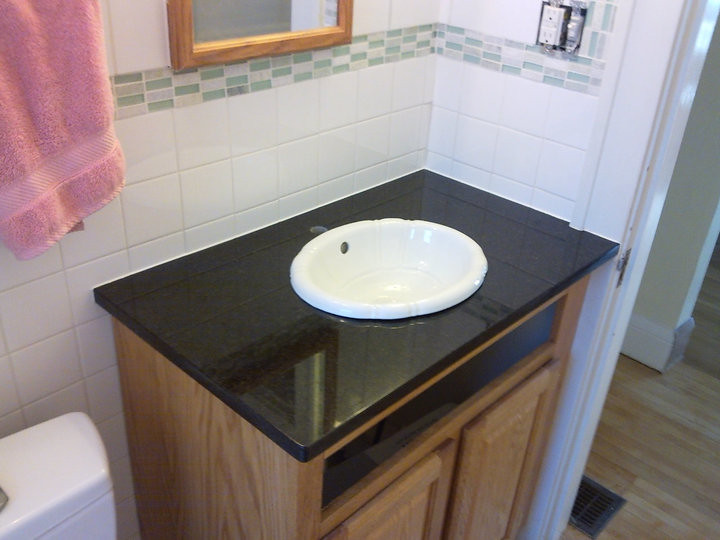The image captures a detailed view of a bathroom. In the bottom left corner, a portion of a toilet is visible. The walls are adorned with tiles; above the toilet hangs a pink, fuzzy towel featuring a smooth stripe pattern. Adjacent to the towel, a brown-framed mirror is mounted on the wall. The wall tiles transition midway to an arrangement of small rectangular tiles in shades of green, white, and speckled with occasional gray and blue.

To the immediate right on the wall, there is an exposed electrical receptacle without a faceplate, revealing the sockets and the gang box. Nearby, a white light switch is also visible. The floor is covered in brown wood, where a floor vent can be seen outside the door, leading to a hallway and another doorway.

The bathroom sink is set in a black marble countertop, distinguished by its small, round, white basin which lacks a faucet and handles. Just below the countertop, there is an open space where a drawer should be, followed by two cupboard doors on a wooden stand.